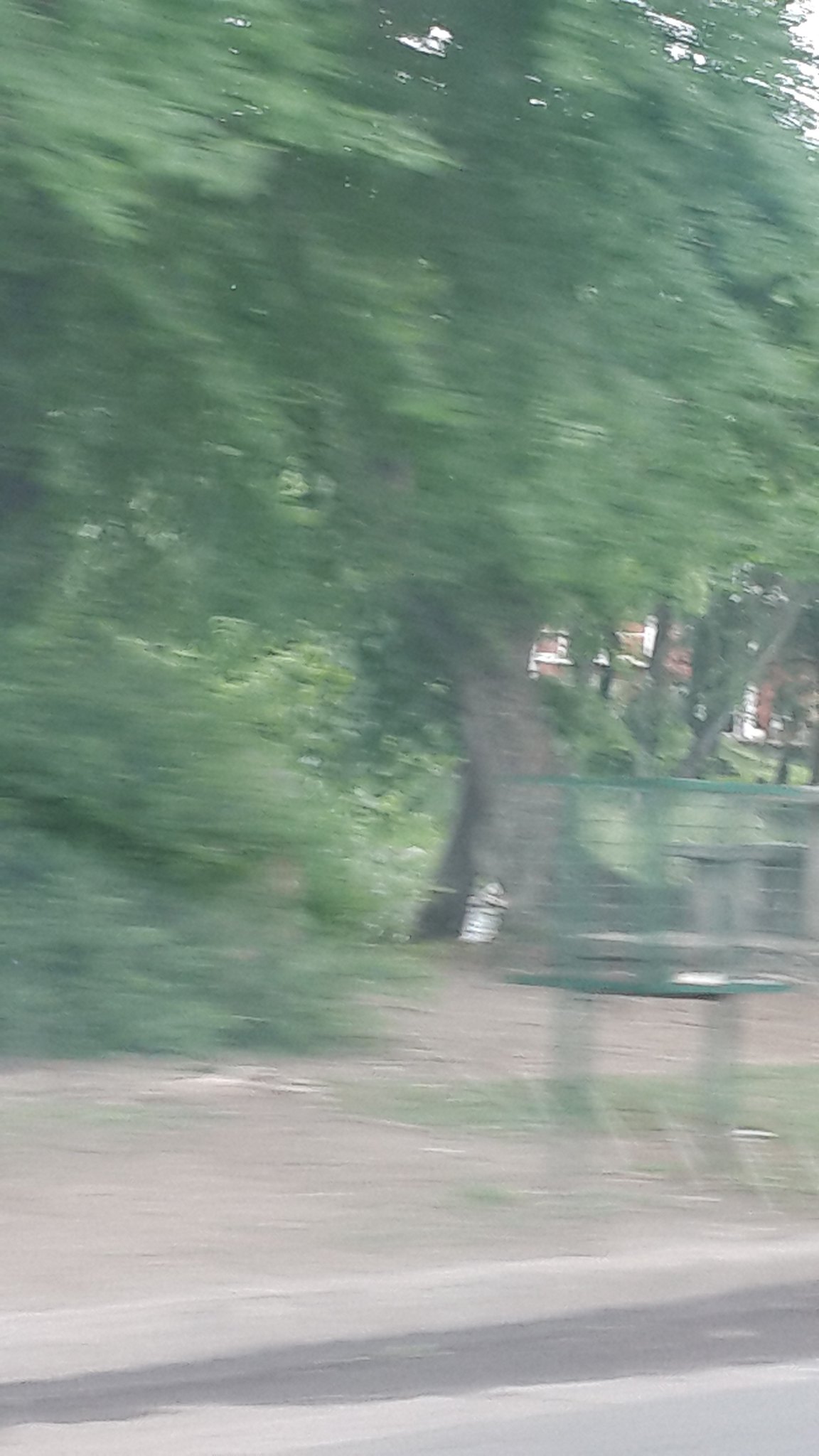A vertical-oriented photograph likely taken from a moving car, evident by the pronounced motion blur and a faint glimpse of the road at the bottom. Dominating the center of the image is a towering tree with a thick, brown trunk, its upper reaches adorned with lush green leaves and foliage. To the right bottom corner, partially obscured by the motion blur, is an indistinct object that could be a bench or a sign, adding an element of mystery. The roadside dirt patch emphasizes the transient nature of the scene, captured in a fleeting moment of travel.